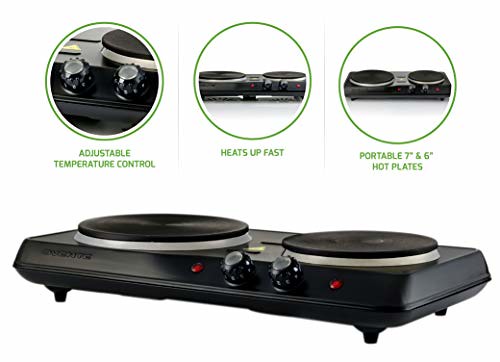This image displays a double burner hot plate with a sleek black rectangular base supported by short legs. The hot plate features two black control knobs with silver tops, positioned symmetrically on the front, each accompanied by a red light indicator. Each burner is adorned with silver bands, supporting flat black tops, approximately the size suitable for a standard plate.

Above the main image are three additional illustrations, each encased in green circles and isolated by thin gray lines. The first illustration shows the two control knobs and highlights the adjustable temperature control with text below. The adjacent illustration offers a front-on perspective of the hot plate, emphasizing rapid heating capabilities, with "heats up fast" written underneath. The third circle presents a slightly angled view, pointing out the portable nature of the 7-inch and 6-inch hot plates, as indicated by the accompanying text.

In the main image, additional details include a partially visible yellow warning triangle with a black line beneath it and the presumed brand name "Ignite." This comprehensive layout showcases the functional elements and user-friendly features of the double burner hot plate, making it an ideal choice for portable cooking needs.